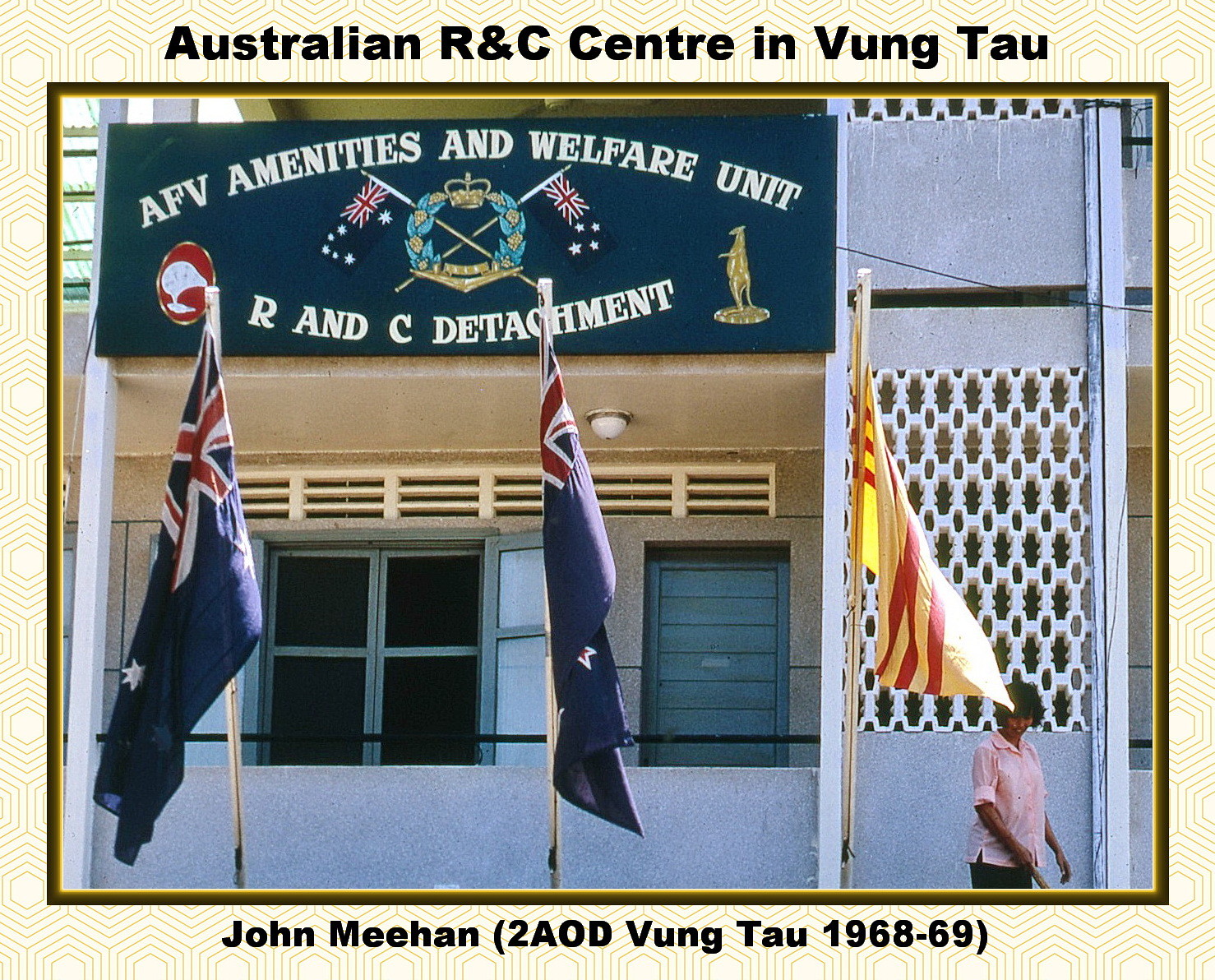This photograph depicts the Australian R&C (Rest and Convalescence) Center in Vung Tau. Prominently displayed are three flags in front of the building: two British flags on the left, characterized by their navy blue color with red and white stripes, and an unidentified third flag on the right with yellow and red colors. The image features a navy blue background sign that reads "AFV Amenities and Welfare Unit, R&C Detachment." A woman, appearing to be in her 30s or 40s, walks behind the flags. At the bottom of the photograph, text states "John Meehan, (2AOD) Vung Tau, 1968-1969." The overall scene suggests a historical setting from the late 1960s.